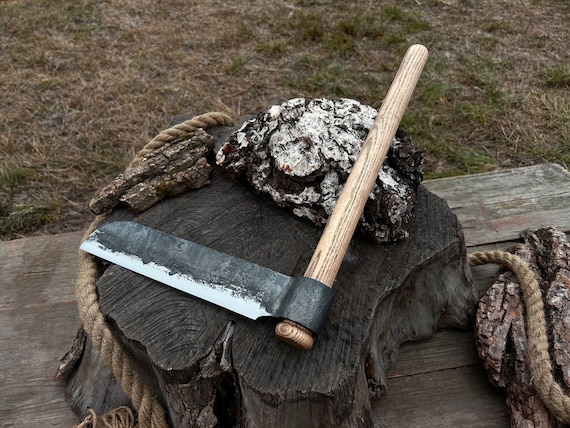The image captures an unusual axe positioned on a dark brownish-gray tree stump. The photograph is taken from an overhead angle, emphasizing the smooth cut of the tree stump, which now serves as a makeshift table or platform. The axe, with its unique design, features a long, curved wooden handle extending diagonally to the right. Its blade, a striking combination of dark gray and silver, extends horizontally across the handle, resembling a large knife or sword more than a conventional axe. The blade has a sharp edge along the center and a blunt edge towards the bottom.

Adjacent to the axe is a prominent light brown rope, which loops around the stump and extends off to the bottom right corner of the image. Additionally, there appears to be a piece of wood or rock with white markings, possibly indicative of mold, resting on the tree stump near the axe handle.

The background reveals a wooden deck or patio that surrounds the stump, creating a rustic atmosphere. Beyond the deck, a patchy yard comprising a mix of brown and green grass adds a natural yet slightly neglected touch to the scene.